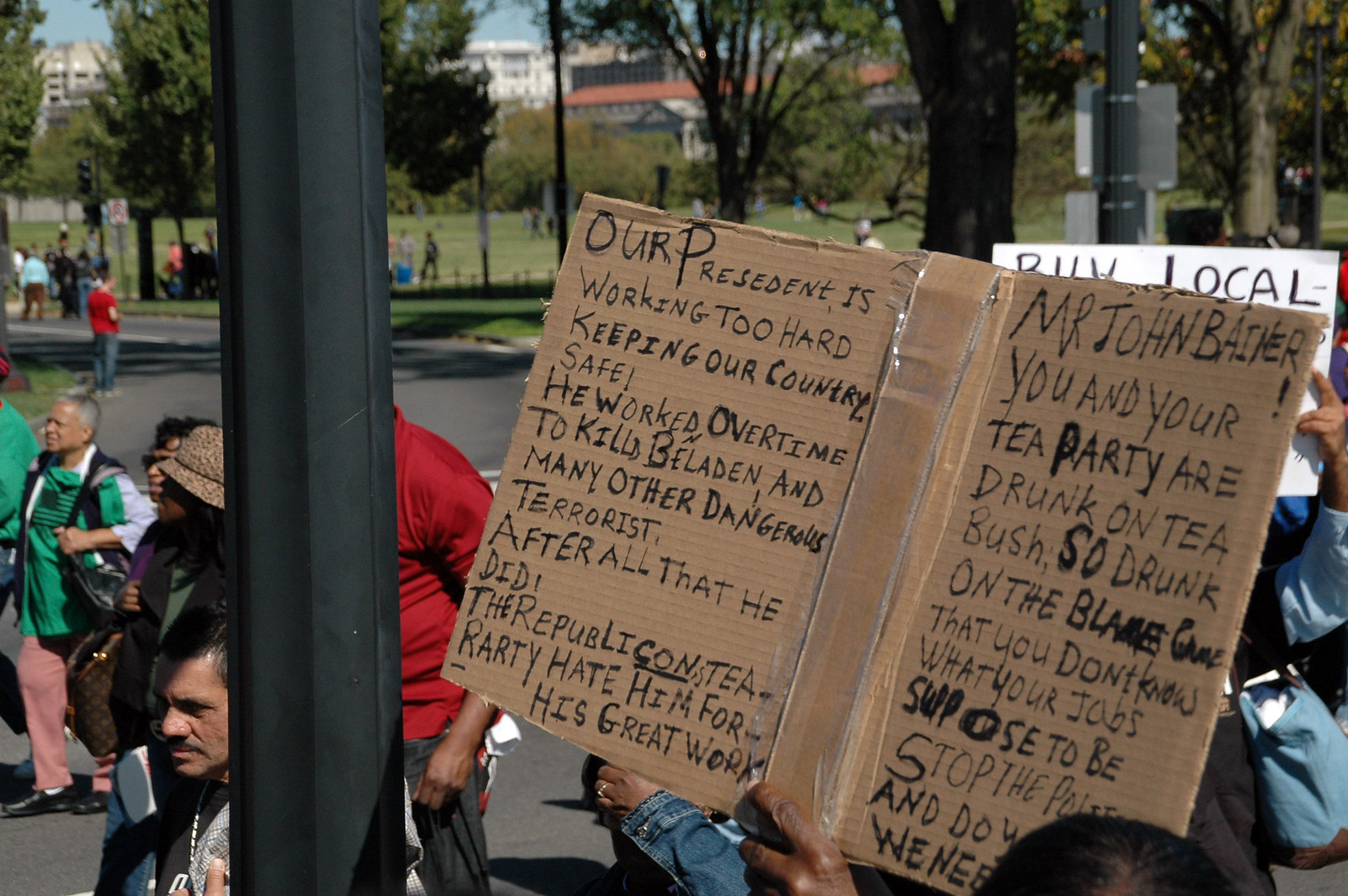In an open outdoor setting under blue skies, a large group of people gather for what appears to be a protest or demonstration. The scene is vibrant with hands raised, holding homemade signs, indicating a collective expression of opinion. At the forefront of the crowd, a man prominently displays a brown cardboard sign, sloppily written in black marker. Despite its hasty penmanship, the sign conveys a clear message: "Our president is working too hard, keeping our country safe. He worked overtime to kill Bin Laden and many other dangerous terrorists. After all that he did, the Republican Tea Party hates him for his quick work. Mr. John Boehner, you and your Tea Party are drunk on T. Bush. So drunk on the blame game that you don't know what your job's supposed to be."

While part of the sign is obstructed by the heads and hands of the crowd, and a black pole blocks some faces, the fervor of the demonstrators is palpable. Behind the crowd, trees provide a lush backdrop, partially obscuring distant buildings. The atmosphere is charged with emotion as people unify to voice their opinions.